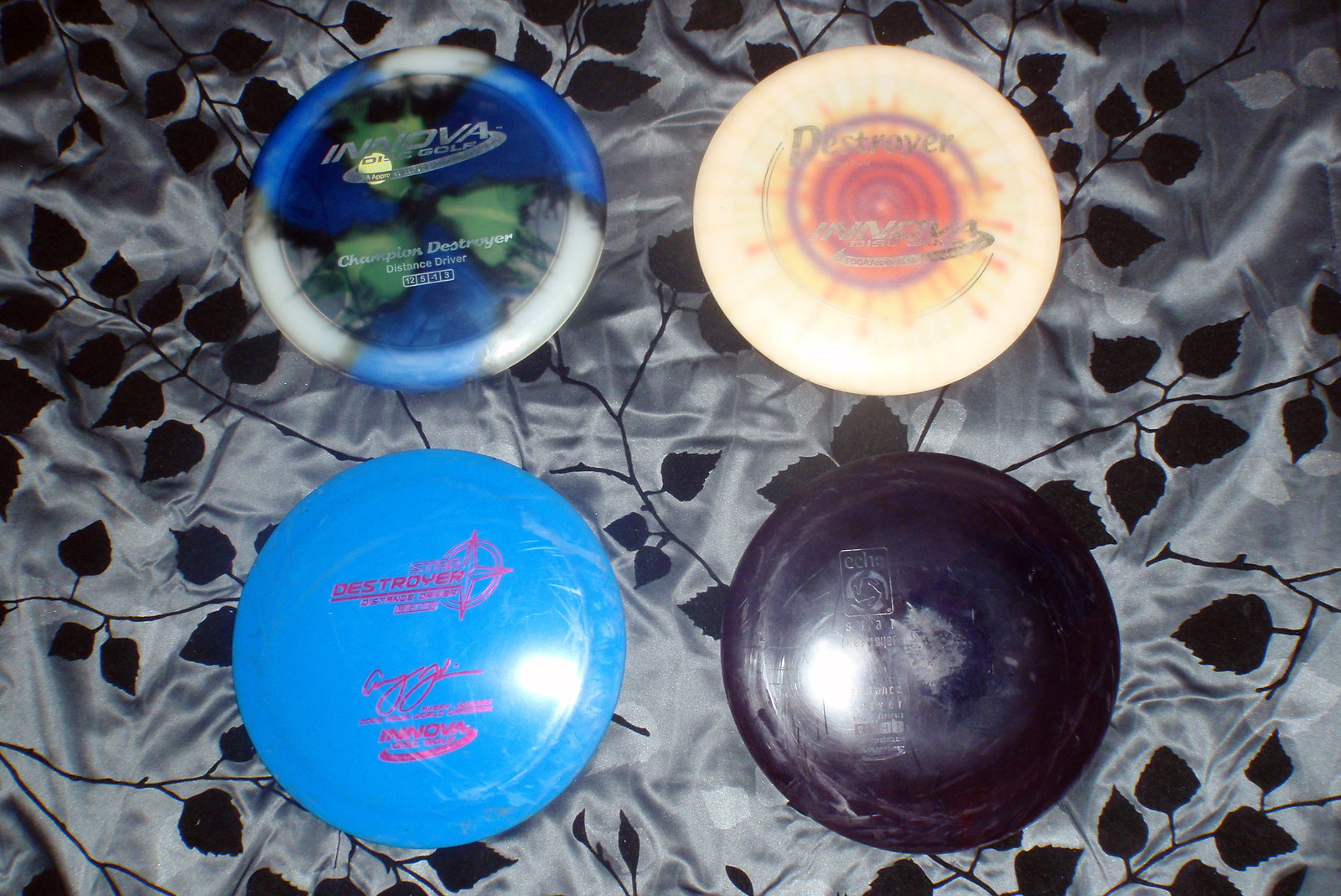The image shows a photograph taken from above, capturing four colorful discs likely used for disc golf, arranged on a gray blanket with an embroidered black leaf and branch design. The top left disc is tie-dyed in white, blue, green, and black colors and has silver text that reads "Innova Disc Golf" at the center, with "Champion Destroyer Distance Driver" and the numbers "12 5 -1 3" underneath. The top right disc features a vibrant tie-dye pattern resembling the sun with colors of purple, orange, and yellow. It also has the "Destroyer" label. The bottom left disc is a solid teal blue with pink text stating "Destroyer Distance Driver" along with a small star logo. The bottom right disc is black, displaying some scratches and is partially obscured by camera flash glare, making its markings less readable. The entire setup is placed on the detailed patterned blanket, adding a textured backdrop to the dynamic array of the discs.